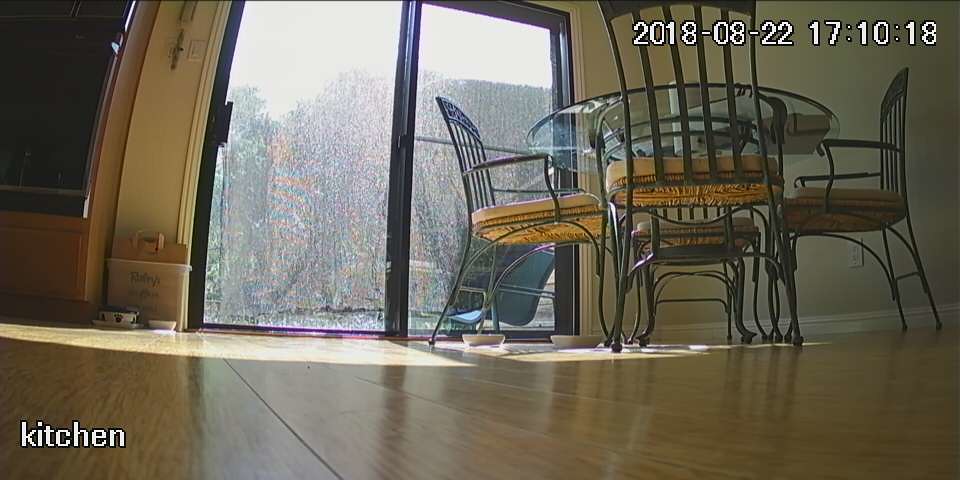Captured by a ground-level security camera with a subtle fisheye effect, this image offers a comprehensive view of an indoor setting. The focal point of the shot is a kitchen area, featuring a glass patio sliding door that allows natural light to filter in. The floor is composed of rich, polished wood, adding a warm touch to the scene. Dominating the room is a glass-top kitchen table surrounded by elegant wrought iron chairs with tan cushions, creating a sophisticated yet cozy dining space. The bottom corner of the image bears the label "kitchen," confirming the room's purpose. Additionally, a time stamp displayed at the top reads "2018-08-22, 17:10:18," indicating the exact moment this snapshot was taken.